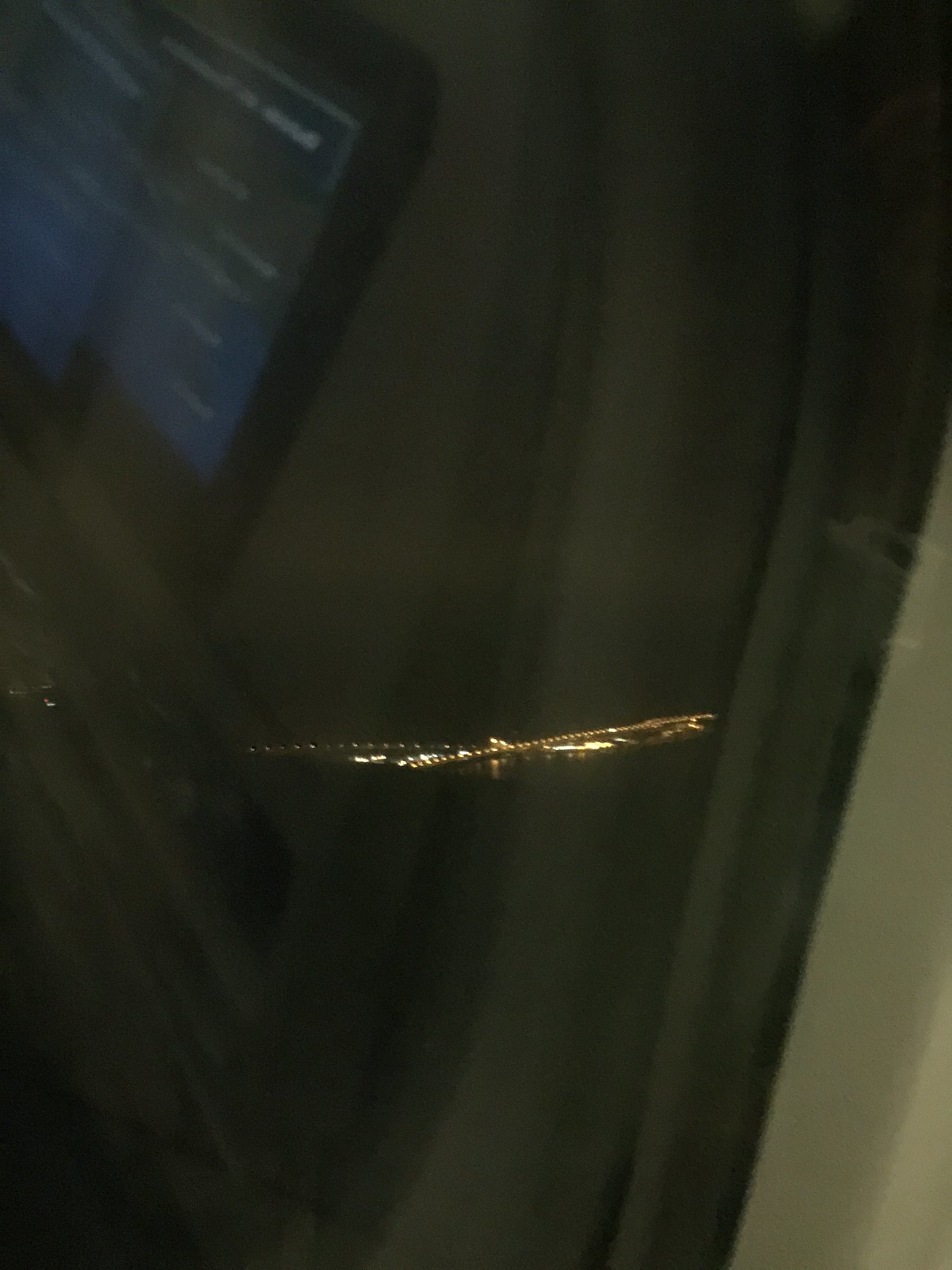The image depicts what appears to be the interior of a device or vehicle, characterized by a predominantly gray color scheme. Central to the image is a screen with a peculiar visual effect resembling double vision—the primary screen is flanked by a secondary, slightly offset projection to its left. The screen features a central line of a gold hue, reminiscent of a scratch. The right side of the image displays a light gray background, contrasting with darker gray areas enveloping the rest of the scene. In the upper left corner, there is a black, square-shaped boundary encasing a screen that is divided into a blue and black half, adorned with white text. This elaborate arrangement suggests a complex, possibly high-tech environment, though its specific function remains uncertain.